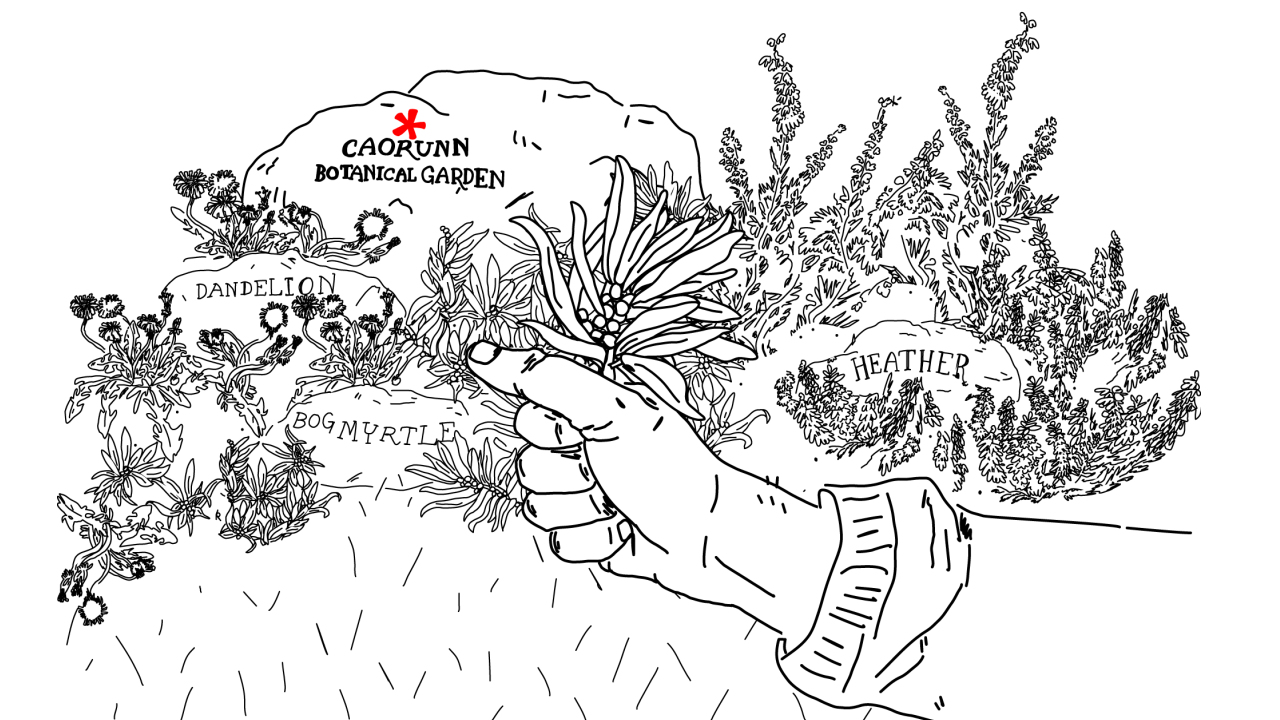A black-and-white stencil drawing showcases a detailed scene with a white background. At the center, a hand emerges from the bottom right corner, holding a small plant with berries. The hand's sleeve is slightly pulled back. Surrounding this central figure are various plants and rocks. To the right of the hand, the word "Heather" is inscribed on a rock amidst the plants. To the left, another rock is labeled "Bog Myrtle," and further to the left, a third rock is marked "Dandelion," each surrounded by their respective flora. In the background, there is a larger rock with the inscription "Caorunn Botanical Garden" in black ink, and atop this rock is a red asterisk. The entire illustration is rendered in a pencil-like style, emphasizing the fine details and textures of the vegetation and rocks, except for the singular red asterisk, which provides a pop of color in the monochrome setting.